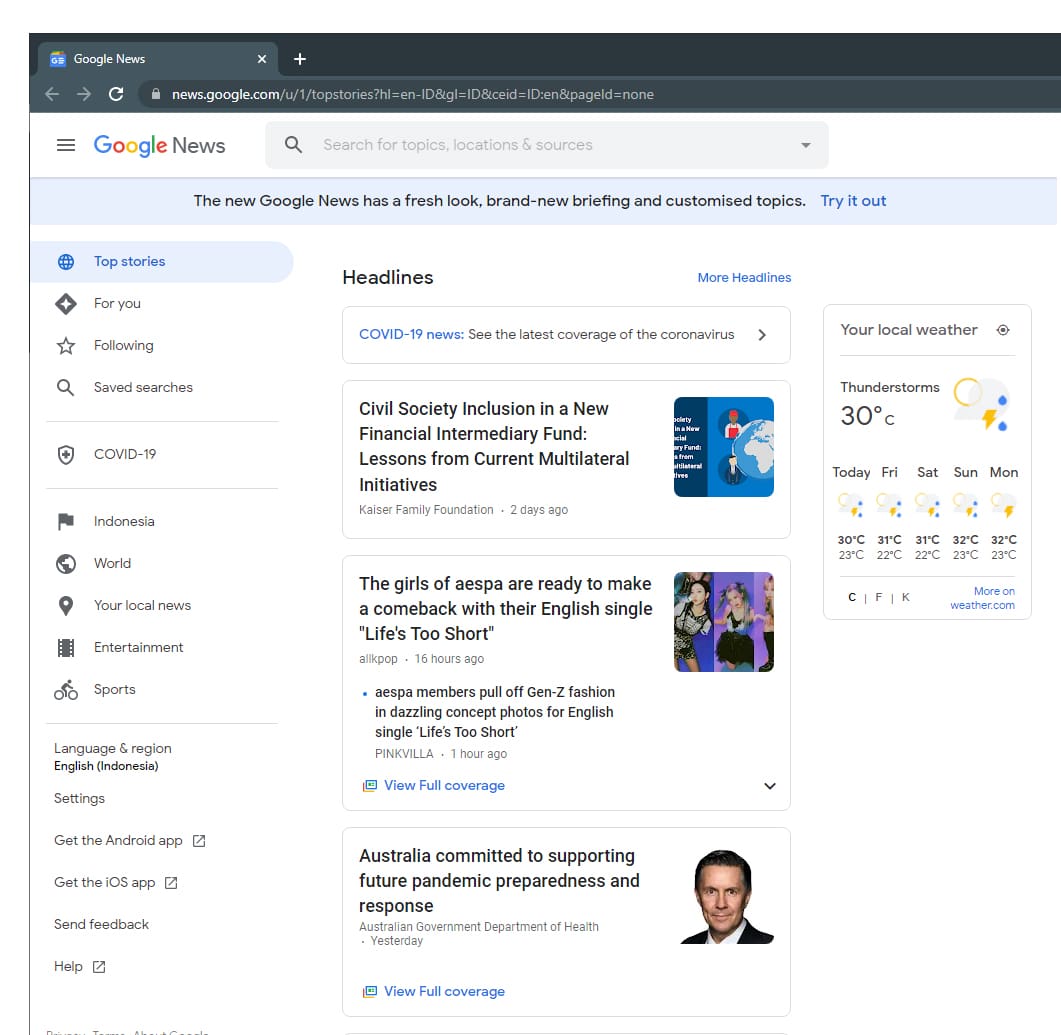The image showcases a Google News webpage with a detailed layout. At the very top, there's a black navigation bar. On the left side of this bar, the words "Google News" are displayed in white. Next to it, there's a white "X." To the right of the "X," there's a plus sign for adding a new tab. 

Below this navigation bar, on the far left, there are left-facing and right-facing gray arrows. Next to these arrows, there's a white refresh button. On the far right, a gray lock icon precedes a URL that reads: news.google.com/u/1/top stories?hl=en-ID&gl=ID&ceid=ID:en&pageId=none.

Underneath this URL bar, on the left side, there are three horizontal black lines stacked vertically, indicative of a menu. To the right of this menu icon, the words "Google News" are displayed once more. In the middle of the page, there is a search bar. 

Further down, a light blue rectangular bar announces, "The new Google News has a fresh look, brand new briefing, and customized topics" in black text. To the right, a clickable text reads "Try it out" in blue.

On the left side of the page, a column lists different sections. At the top, "Top stories" is highlighted in blue. Below that, an image of a diamond signifies the "For you" section, labeled in gray. Under that, a star signifies the "Following" section, also in gray. A magnifying glass icon marks the "Saved searches" section, and a shield with a plus sign indicates the "COVID-19" section, both in gray. Further down, icons such as a flag (Indonesia), a globe (World News), a location marker (Your local news), a film strip (Entertainment), and an outline of a cyclist (Sports) are displayed, all in gray.

In the main content area, the section heading "Headlines" is in black. Directly under it, "COVID-19 news" is highlighted in blue with a prompt to "See the latest coverage of the coronavirus" followed by a right-facing arrow, all in gray.

The headlines begin with a news story titled "Civil Society Inclusion in a New Financial Intermediary Fund: Lessons from Current Multilateral Initiatives" in bold black letters. It is attributed to "Kaiser Family Foundation," dated two days ago in gray.

Another headline reads, "The girls of AESPA are ready to make a comeback with their English single Life’s Too Short" in bold black letters. Beneath it, "ALLKPOP" is noted, with the timestamp "16 hours ago" in gray. A sub-headline below states, "AESPA members pull off Gen Z fashion and dazzling concept photos for English single Life’s Too Short," followed by "Pink Villa" and "one hour ago" in gray. To the left of this headline, a blue clickable text reads, "View full coverage."

Further down, a headline states "Australia Committed to Supporting Future Pandemic Preparedness and Response" in bold black letters. This is attributed to the "Australian Government Department of Health," dated "yesterday" in gray. Under it, "View full coverage" appears again in blue. To the right of this news headline, there's an image of a man with short dark hair and tan skin.